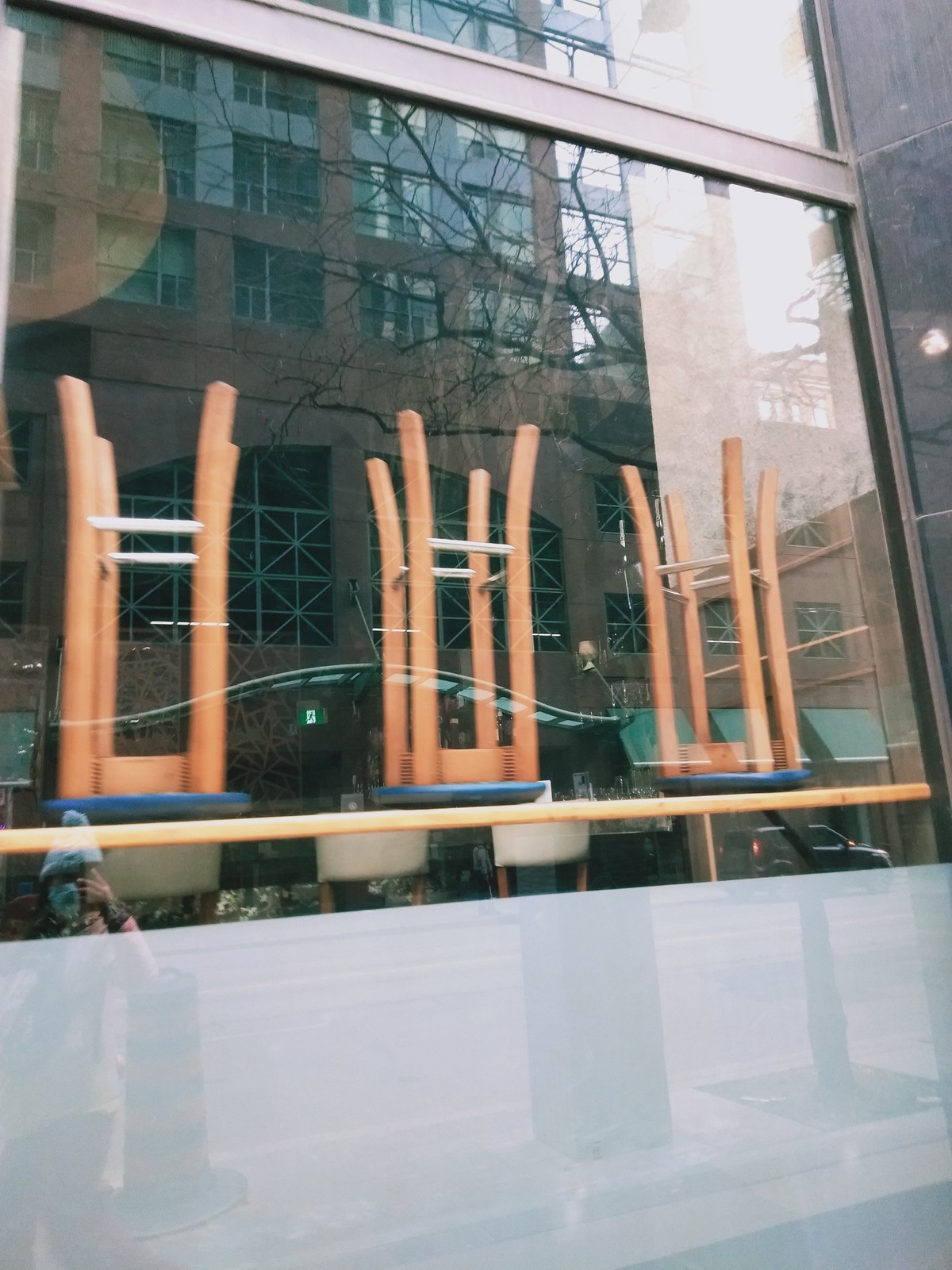This photograph captures the exterior of a commercial building and looks through its large plate glass windows into what appears to be a closed business, likely a coffee shop or restaurant. Inside, a counter or bar runs along the window with three blue-topped stools turned upside down on the countertop, indicating that the establishment is not currently open. The building is tall, and in the window’s reflection, you can see the photographer—a woman wearing a hat and a mask—which suggests this picture might have been taken during the COVID-19 pandemic. Her reflection is alongside the reflection of a neighboring building with a couple of awnings, as well as a car, hinting that the setting is likely in a downtown area of a city. The window features a white filter at the bottom, transitioning to clear glass on the upper portion, with stone detailing visible on the building itself.